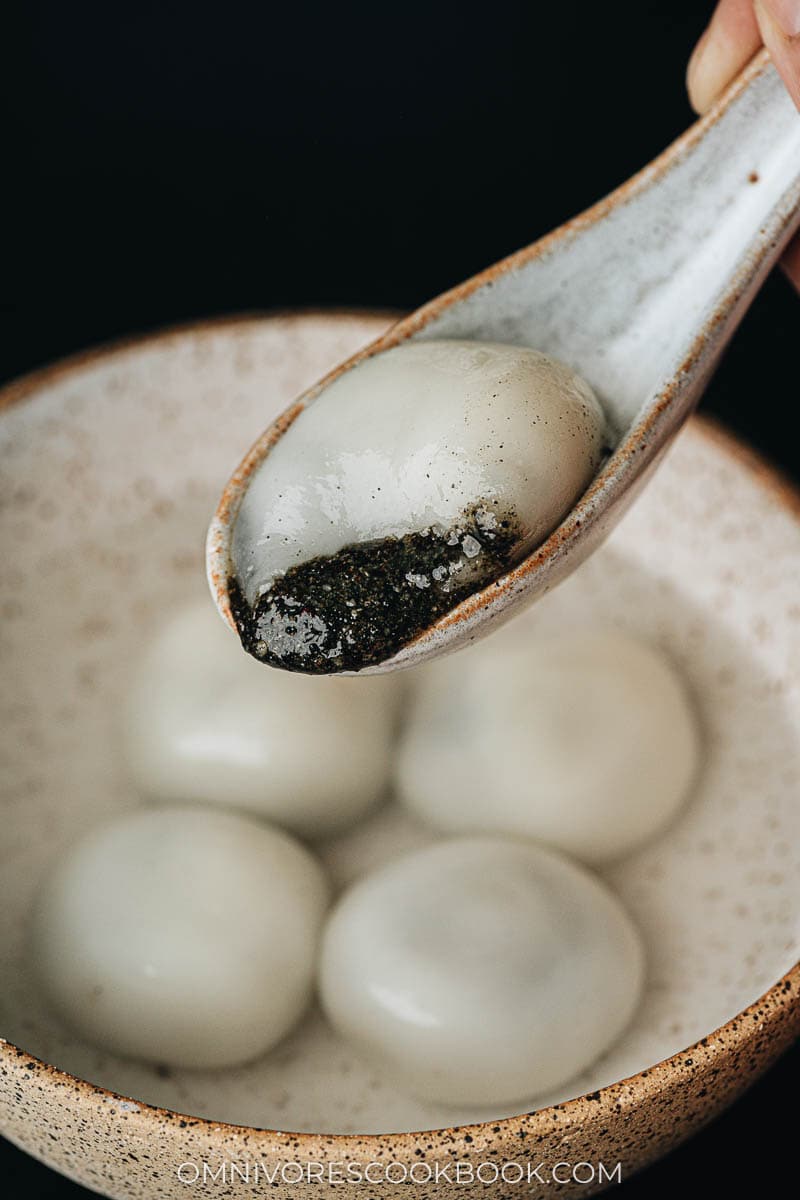The photograph is a detailed and realistic food image showcasing a ceramic bowl filled with four white dumplings, each intricately speckled with brown patterns. The bowl, prominently placed at the center of the image, features an orange and white exterior with black speckles, and a beige interior similarly speckled. The bowl is half-filled with water, in which the dumplings float, softening the focus of those below the water surface. A matching ceramic spoon, held by a person, hovers above the bowl, cradling a fifth dumpling that is partially open, revealing a rich black sesame filling that oozes slightly. The overall background of the photo is a stark black, enhancing the clarity and color of the subject. At the bottom of the image, the website omnivorescookbook.com is clearly displayed in white text. The image, in portrait orientation, blends the aesthetics of photographic realism with food photography to draw attention to the dish, likely meant as a recipe feature.